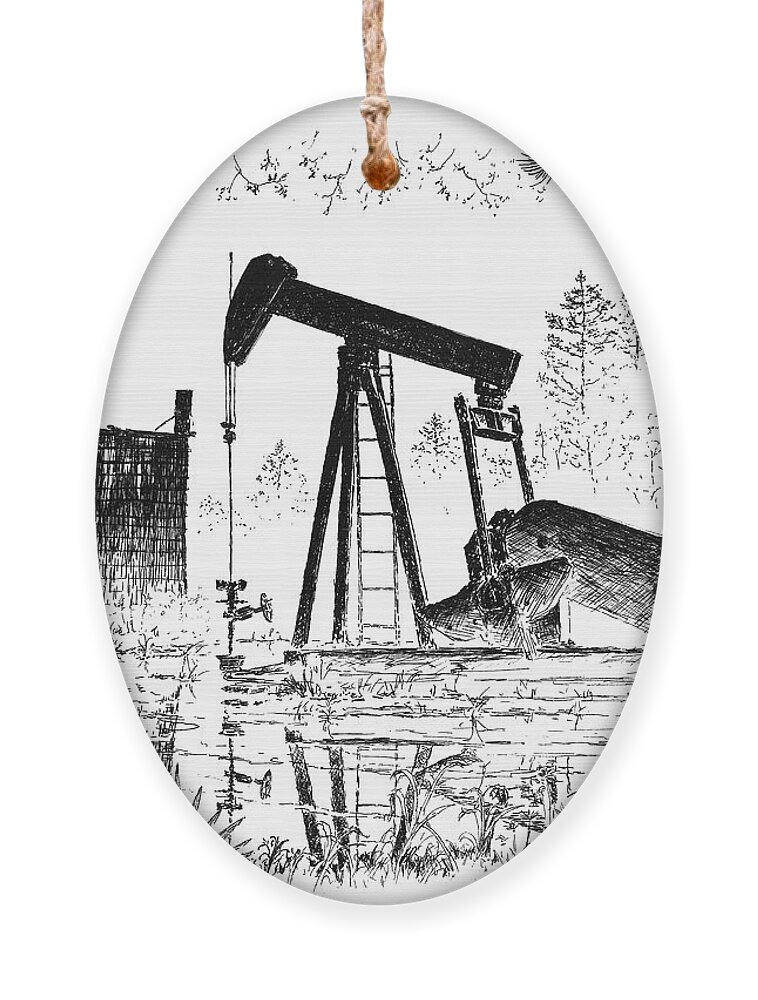This detailed black and white illustration, encased in an oval pendant with a brown rope for hanging, depicts a historic rural scene. Central to the image is an old-fashioned drilling machine working on the ground, detailed in pencil-like strokes. To the left stands a modest house, possibly wooden, accompanied by a surrounding fence. In the foreground and background, various crops and flowering plants are depicted, alongside a collection of trees, lending a pastoral quality to the scene. Above the pendant, three branches and part of the hanging rope are visible, suggesting it could be displayed as a necklace or decor. The entire composition is reminiscent of an old, nature-focused engraving with intricate details capturing a serene, rural landscape juxtaposed with early industrial activity.